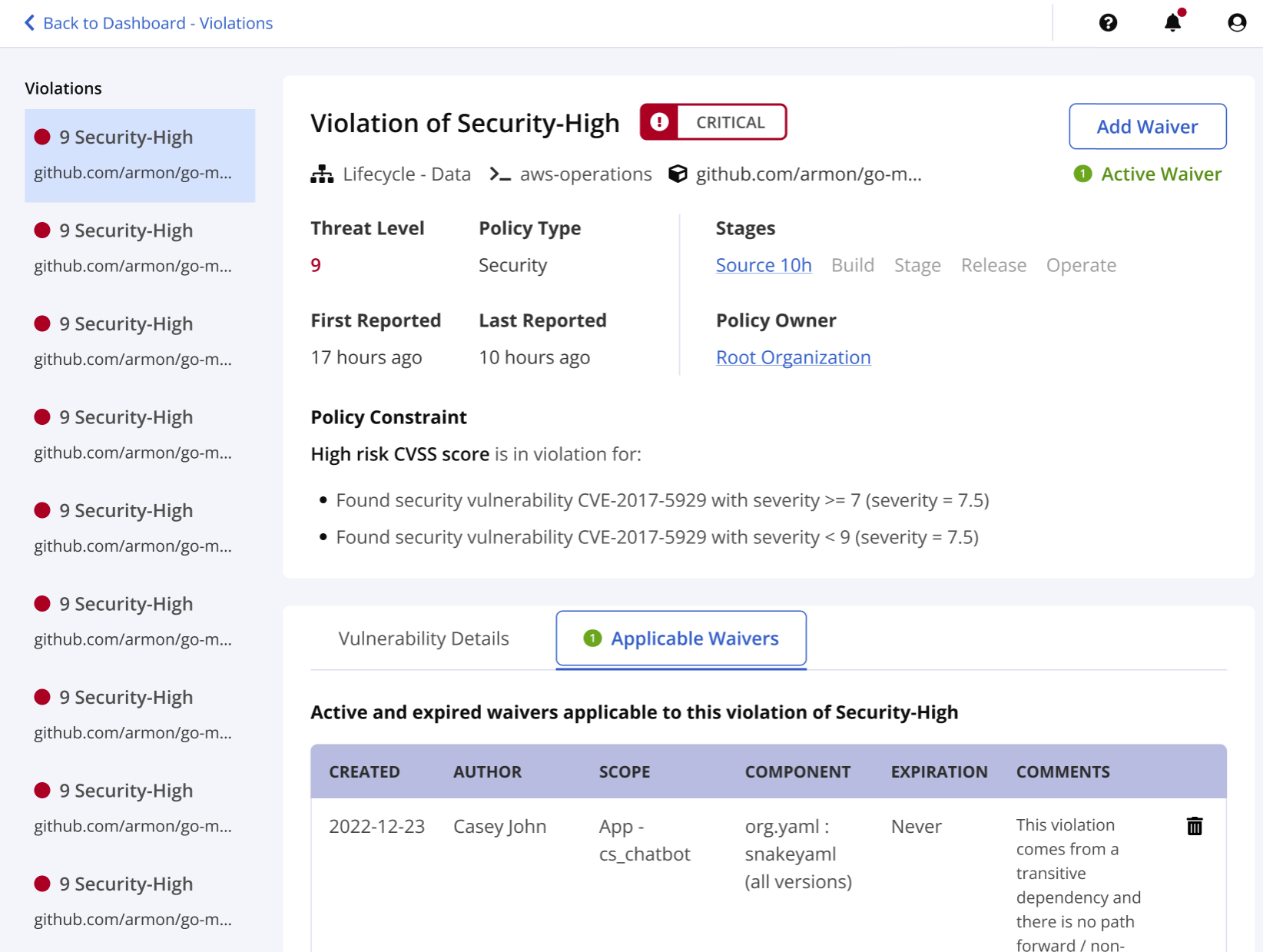The image displays a user interface for monitoring security violations within Amazon Web Services (AWS). At the top, there is a navigation option labeled "Back to Dashboard," indicating the current focus on the "Violations" section. On the left side, a list of "Security High Violations" is visible, with multiple entries that appear uniform. On the right side, detailed information for a selected violation is presented. This particular violation is classified as "Security High" and marked critical, with a threat level of nine. The policy type is labeled as "Security," and the policy constraint specifies "High-risk CVSS scores." The violation details indicate that there were four security vulnerabilities found, with one scoring around seven and another slightly less than nine on the CVSS scale. The section further down the page provides additional vulnerability details and information about applicable waivers. The interface seems to cater to technical professionals familiar with cybersecurity metrics and AWS protocols.